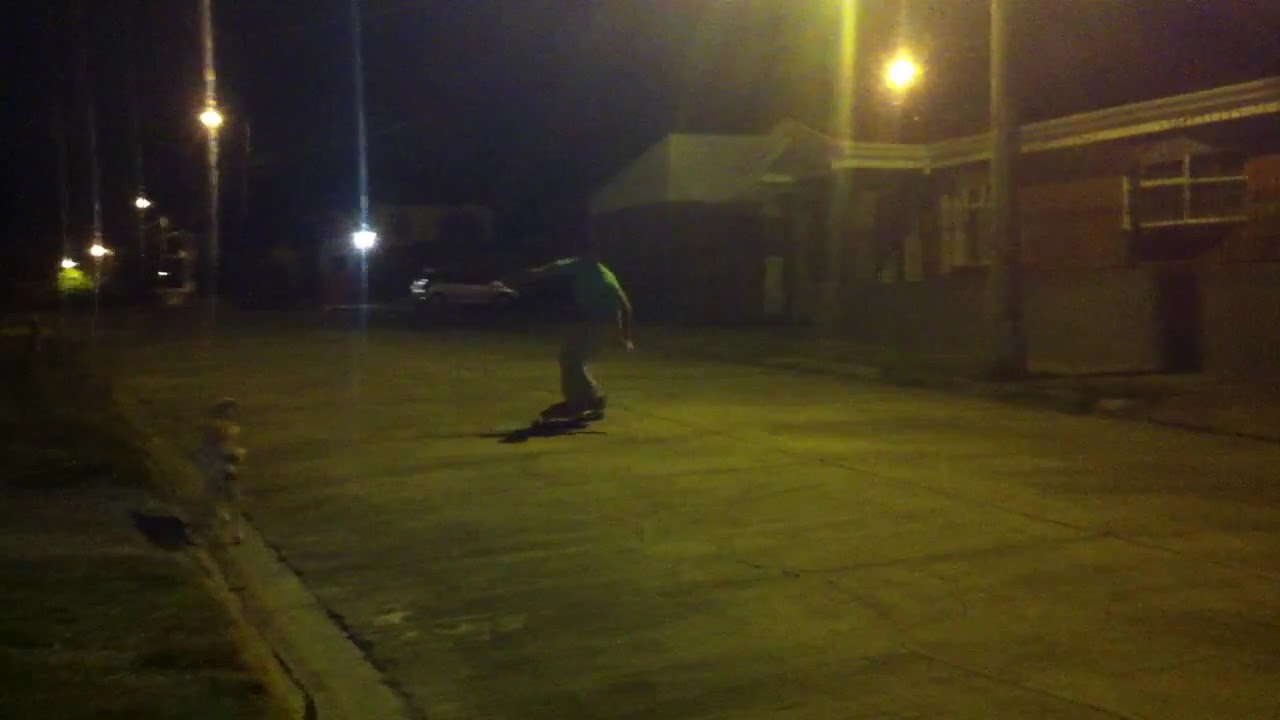In this nighttime scene, a young man is captured skateboarding down a dimly lit residential street, illuminated by six street lamps. He wears a green short-sleeved shirt and light-colored pants, extending his arms out slightly for balance. The street, which is dry and devoid of rain, features a fire hydrant to the left of the skateboarder, nestled alongside a patch of grass. To the right, there's a one-story red brick building with a white roof, possibly an office or an apartment building. Behind the skateboarder, in the background, are more residential houses and buildings, partially obscured by darkness. A silver car is parked on the road facing right, adding to the depth of the scene. The streetlamps cast a soft, ambient glow, highlighting the skateboarder's path and subtly illuminating the surroundings.